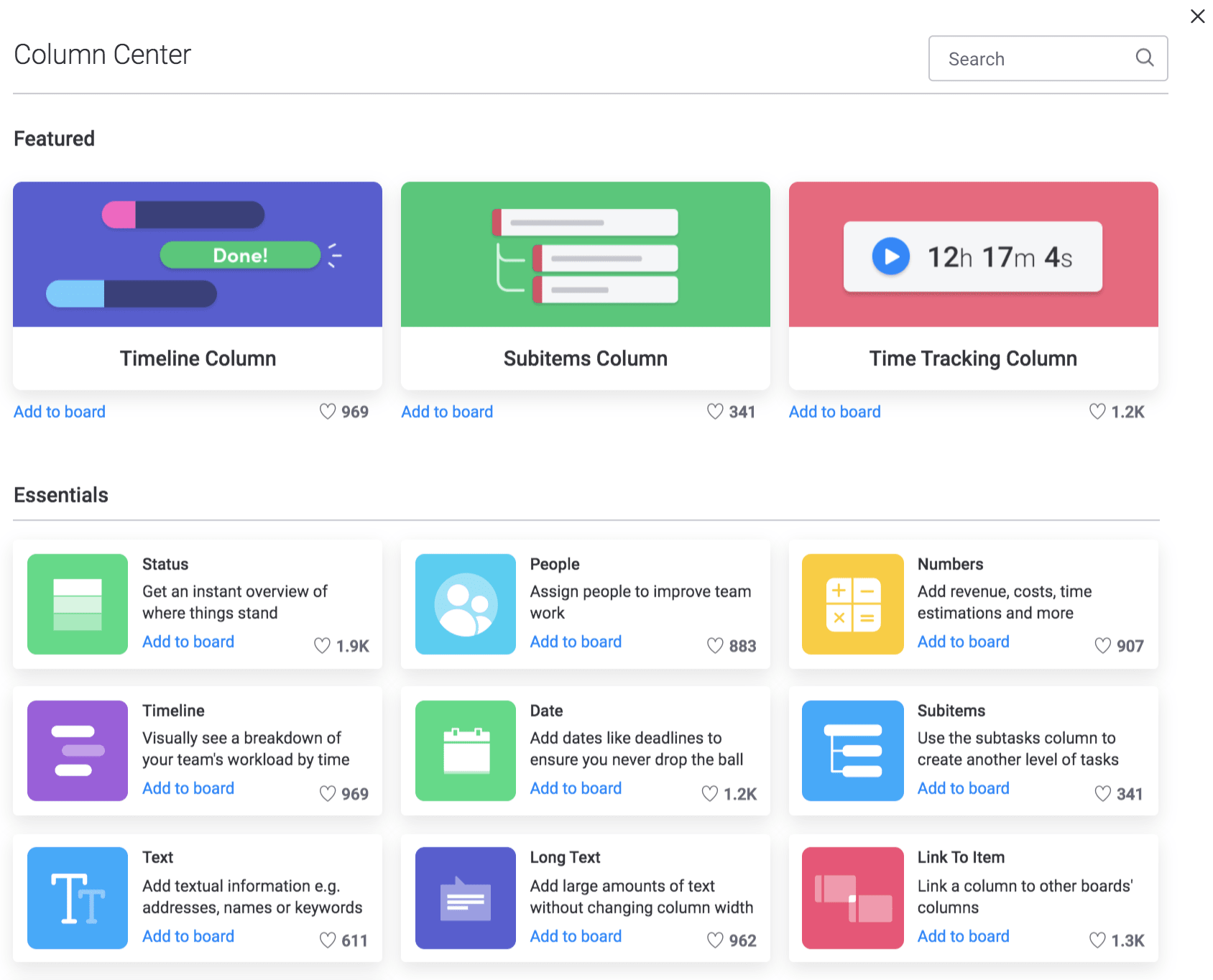This image depicts a computer screen displaying a webpage with a section titled "Column Center" at the top in black text. On the far right of this row, there is a search box featuring the word "Search" accompanied by a magnifying glass icon and an 'X' in the upper right-hand corner.

Below this section, there is a header labeled "Featured" under which three distinct rectangles are displayed. The first rectangle is purplish and contains various smaller rectangles inside. One of these smaller rectangles includes the word "Done" in green text and another label reading "Timeline Column." Adjacent to this, in the center, is a green rectangle that resembles sticks of dynamite and has the label "Sub-Items Column." The third rectangle, situated to the right, is outlined in pink and features a blue play button with a timer indicating "12 hours, 17 minutes, 4 seconds," labeled as the "Time Tracking Column."

Each of these featured rectangles includes a prompt that allows the user to "Add to Board" in blue text, accompanied by a heart icon for liking the content.

Below the featured section is an "Essentials" area, consisting of three rows, each containing three rectangles: in the first row, a green box labeled "Status," a blue box labeled "People," and a yellow box labeled "Numbers." The second row includes a purple box labeled "Timeline," a green box labeled "Data," and a blue box labeled "Sub-Items." The third row features a blue box labeled "Text," a purple box labeled "Long Text," and a pink box labeled "Link to Item."